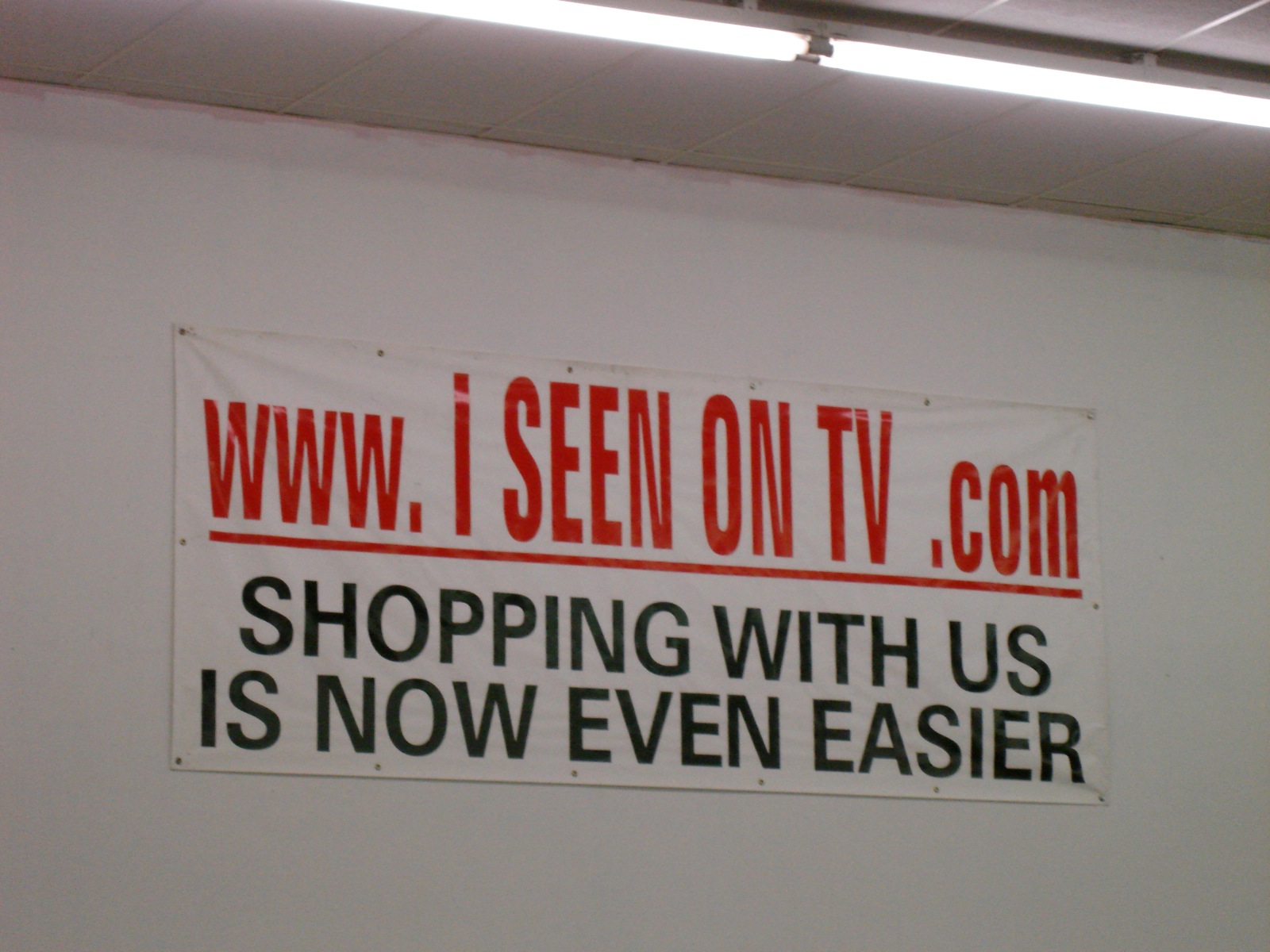In a warehouse-like indoor shopping venue, a white roll-up banner is pinned to a white wall using multiple tacks—six along the top, six at the bottom, and one on each side in the middle. The banner prominently showcases large red text at the top that reads "www.iceenontv.com." Below this in green capital letters, it declares "Shopping with us is now even easier." Above, fluorescent lights, suspended from a black pipe-like structure, extend diagonally from the upper right corner to just past the left center of the image, casting a utilitarian glow over the scene.